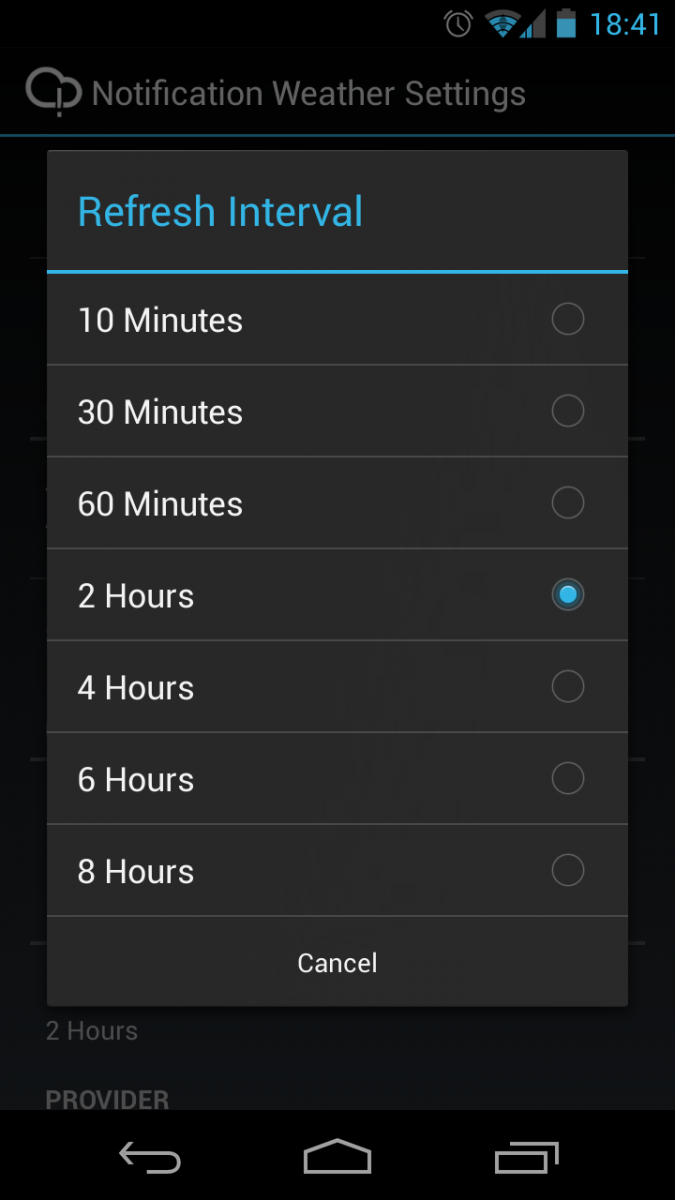The image is a screenshot of a mobile application interface displaying various notifications and settings. At the top-right corner, there are several status indicators: an alarm clock icon, a Wi-Fi signal with three out of four bars, a cellular signal with two out of four bars, and a vertical battery life indicator showing over 70% charge. The time is presented in a 24-hour format as 18:41.

Below these indicators is a warning notification from a weather service, represented by a cloud icon with an exclamation mark inside. This is followed by the weather notification settings. The refresh interval setting is highlighted in blue text, indicating the user can choose their preferred update frequency from the available options listed below.

There are seven different interval options, of which the middle one (2 hours) is selected, indicated by a check mark. The intervals are listed as follows:
- 10 minutes (unchecked)
- 30 minutes (unchecked)
- 60 minutes (unchecked)
- 2 hours (checked)
- 4 hours (unchecked)
- 6 hours (unchecked)
- 8 hours (unchecked)

Beneath these options is a gray line with the word "Cancel" underneath it. Below this, inactive and in darker gray text, is another "2 hours" label followed by the word "Provider."

At the bottom of the screen, there are three icons: one showing an arrow that loops upon itself pointing to the left, a somewhat crushed house icon, and two overlapping box icons.